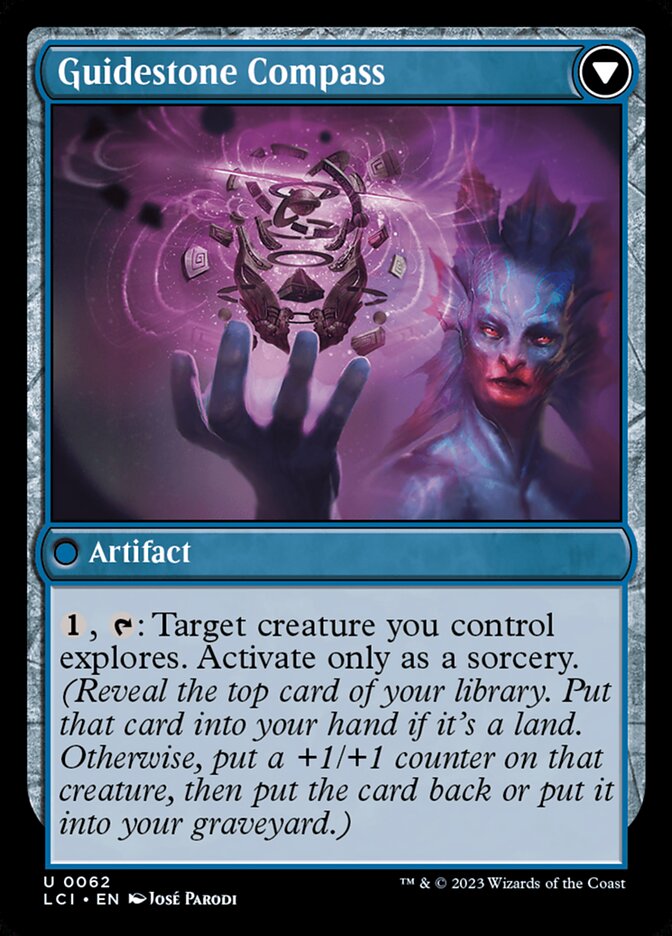This image features a "Magic: The Gathering" trading card titled "Guidestone Compass" from Wizards of the Coast, created in 2023. The card is bordered in black with an interior border that resembles bluish-gray stone. At the top, in a white text, the card name "Guidestone Compass" is written with a white arrow facing downwards. 

The central illustration depicts a bluish-purple amphibian humanoid creature, potentially a merfolk, with fins and pinkish facial features, eyes tinged with red or pink. The creature holds its right hand palm upwards, above which floats a pink and purple artifact. This artifact consists of circles, gears, and various parts, forming a small, swirling galactic sphere.

In a blue box below the image, the card is labeled as an artifact. The text within a lighter blue box reads: "1 Tap: Target creature you control explores. Activate only as a sorcery. Reveal the top card of your library. Put that card into your hand if it's a land. Otherwise, put a +1/+1 counter on that creature. Then put the card back or put it into your graveyard." 

Additional details at the bottom of the card include the identifier "U-0062," the illustrator's name “Jose Parodi,” and the trademark "TM 2023 Wizards of the Coast."